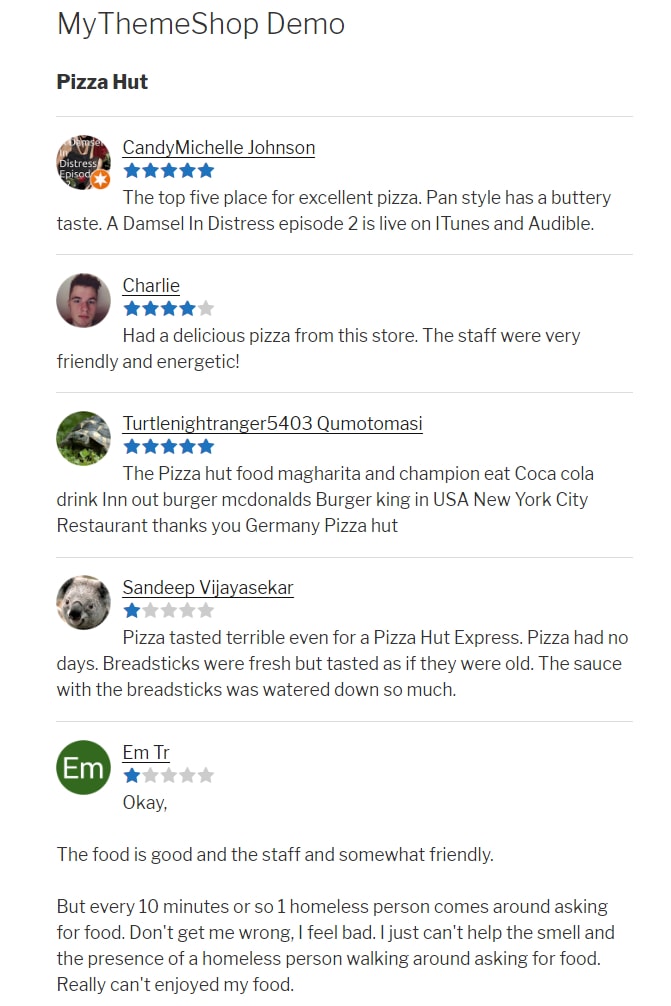Here is a detailed and cleaned-up caption for the image described:

---

This image is a screenshot from the reviews page of a demonstration for "MyThemeShop," a theme design service, demonstrating a theme titled "Pizza Hut." Positioned at the top is the main title "MyThemeShop Demo," with "MyThemeShop" written as a single word. Below, in bold text, is the title "Pizza Hut."

The page features five distinct reviews from various users, each accompanied by their unique avatar or profile picture. Each username is underlined, followed by their star rating, ranging from one to five stars, with a brief corresponding review.

1. **Candy Mitchell Johnson**: 
   - Rating: Five blue stars
   - Review: "The top five places for excellent pizza. Pan Style has a buttery taste. A Damsel in Distress Episode 2 is live on iTunes and Audible."

2. **Charlie**:
   - Rating: Four out of five stars
   - Review: "Had a delicious pizza from this store. The staff were very friendly and energetic."

3. **Turtle Knight Stranger (5403 Kumoto Masi)**: 
   - Rating: Five out of five stars
   - Review: "The Pizza Hut Food Margarita and Champion. Eat Coca-Cola, Drink In-N-Out, Burger McDonald's, Burger Kickin' USA, New York City Restaurant, Thank You Germany, Pizza Hut."

4. **Sandeep Vijayasekar**: 
   - Rating: One out of five stars
   - Review: Negative feedback suggesting dissatisfaction (specific content not provided).

5. **M. Ter**: 
   - Rating: One out of five stars
   - Review: Negative feedback suggesting dissatisfaction (specific content not provided).

The reviews are presented against a white background, each separated by a horizontal line for clear demarcation.

---

This rephrased caption provides a comprehensive and detailed description of the image.